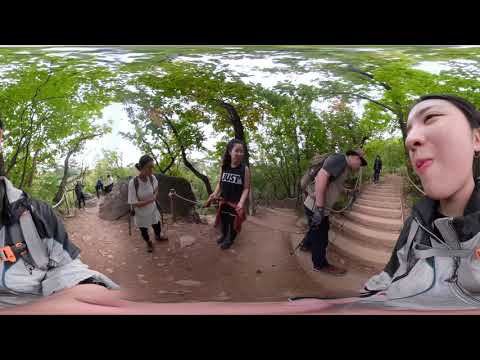A panoramic photograph taken likely with a selfie stick captures an outdoor scene along a developed trail, where a diverse group of young, mostly Asian people, are navigating their way through a distorting lens effect. The trail is lined with concrete or stone stairs, set against a dirt brown ground with scattered stones, surrounded by verdant green trees and the daytime sun. In the foreground, a young Asian woman appears split between the left and right edges due to the panorama's distortion, her playful or sarcastic expression visible. Centered in the midground, a man in a hat, dark pants, and a t-shirt with a backpack prepares to ascend the stairs, accompanied by two young women; one with her hair in a ponytail wearing a black sleeveless shirt with the word "just" on it, and the other with a red shirt tied around her waist. In the far distance to the left, another small group of three hikers is catching up, adding to the dynamic, active ambiance of the scene.